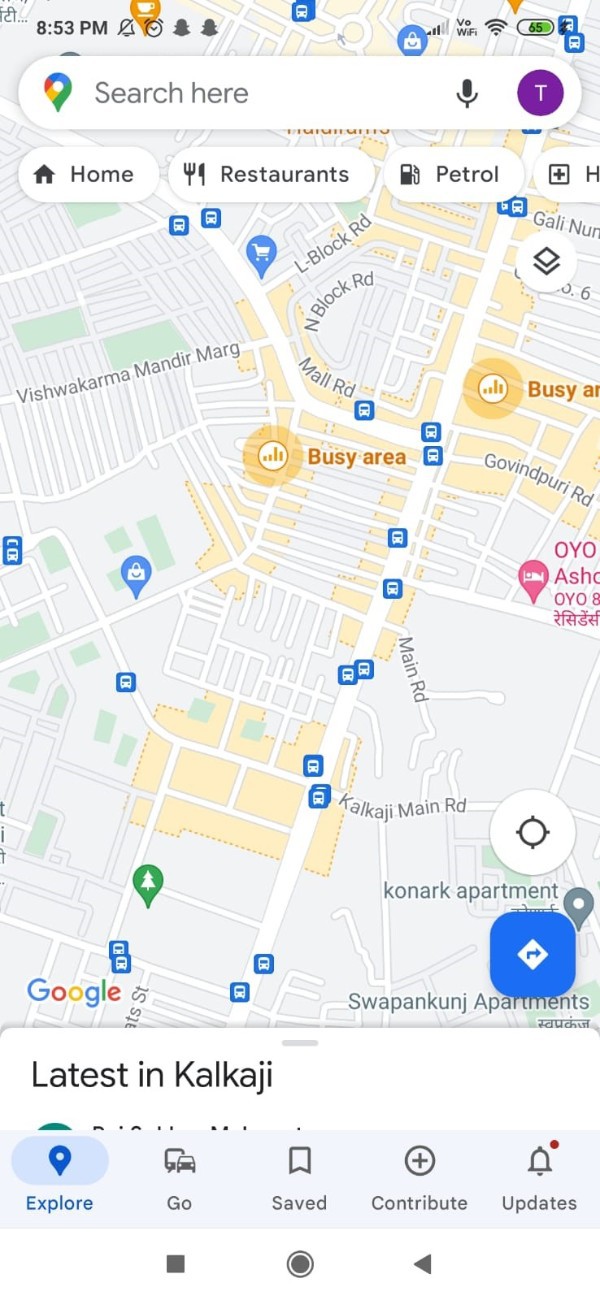A detailed caption for the given image could be:

"The image displays a cell phone screen in portrait orientation, showing a Google Maps interface. At the bottom of the screen, below the map, the words 'Latus' and 'Kalkaji' are visible, with 'Kalkaji' capitalized as K-A-L-K-A-J-I. The interface includes a light bar featuring a blue-highlighted 'Explore' icon and grayed-out options for 'Go,' 'Saved,' 'Contribute,' and 'Updates,' accompanied by a bell icon with a red dot indicating new notifications. 

Further down, there are three primary navigation buttons: a square, a circle, and a left-facing caret. 

The map itself is in color, centered around a yellow circle with the label 'Busy Area' emanating outward. The map features numerous streets, labeled with names such as Vishwakarma Mandir Marj, Elblock Road, Inblock Road, Mall Road, Govindapuri Road, Main Road, Kalkaji Main Road, and Konark. There are also labeled apartment complexes like Konark Apartment and Swapan Kunji Apartments. 

Bus stops are indicated by blue squares with white bus icons, and other icons represent shopping baskets and a bag. At the bottommost part of the map, a blue square with a white diamond and a blue right-facing arrow is visible.

At the top of the screen, the search bar is highlighted, adorned with a colorful Google icon to the left, a microphone emblem, and a blue circle with a 'T' in it. Below the search bar, there are clickable fields labeled 'Home,' 'Restaurants,' and 'Petrol,' directing users to these categories."